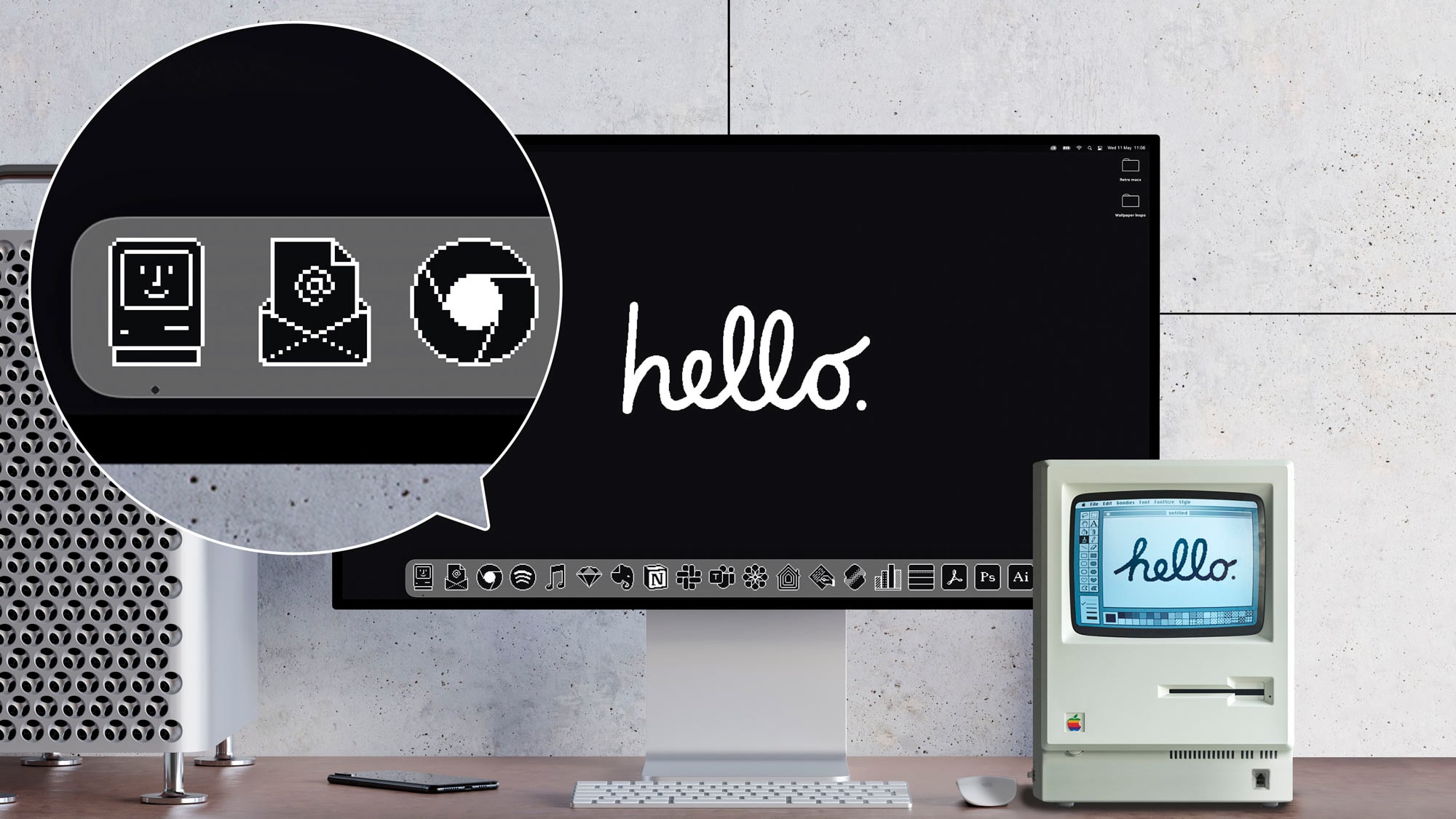The image depicts a detailed setup on a brown wooden desk set against a background of cream-colored or white tile walls forming square patterns. At the center, there is a black rectangular computer monitor with the word "hello." written in white cursive letters. The monitor is supported by a white stand and has a gray taskbar at the bottom displaying various icons, including a computer with a smiley face, an email symbol, and the Chrome logo. In front of the monitor, there is a small white keyboard and an Apple mouse.

To the right of the main monitor, there is an older, boxy computer with a white border and a blue screen that also displays the word "hello." in similar cursive writing. This vintage computer includes a floppy disk drive, emphasizing its antiquity. On the desk, to the left of the main monitor, there is a peculiar, silver grated device reminiscent of a cheese grater, standing on four legs.

Additionally, a phone is lying flat on the desk, contributing to the array of technology showcased in the image. The entire arrangement appears to contrast modern and older technology, potentially suggesting an advertisement or a visual comparison of technological advancements.